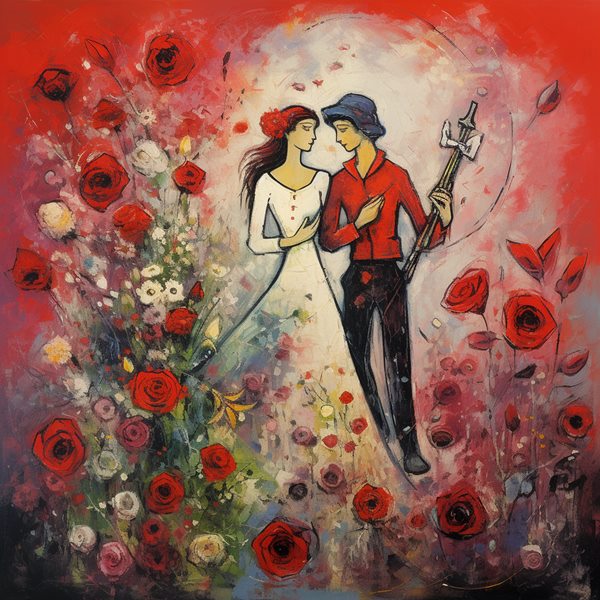The painting features a cartoon-like depiction of a newlywed couple set against a predominantly red background. In the center, standing amidst a vibrant array of red, white, yellow, and pink flowers, the bride, with long flowing brown hair adorned with a red flower, wears a long white dress with a V-neck, exposing parts of her shoulders. Her hair appears to be blowing in the wind, adding a dynamic element to the composition. The groom, standing to her right, is dressed in a red button-up collar shirt, black pants, black shoes, and a blue bucket hat. Their arms are linked together as they face forward and gaze into each other's eyes. The groom holds a sword or scepter-like object in his right hand. Behind them, there is an illusion of a moon created by a whitish-grayish circular area, which enhances the mystical and romantic feel of the scene.